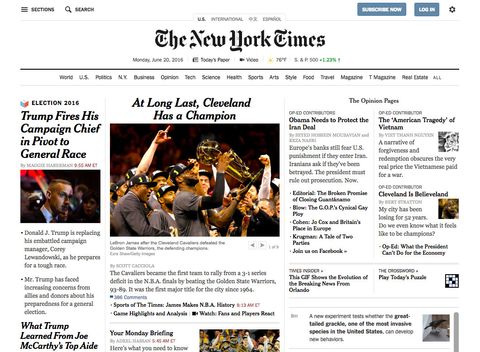The image showcases the front page of the New York Times website. At the top left corner, there is a "Sections" label next to a three-horizontal-line menu icon. Adjacent to this, there is a magnifying glass icon accompanied by the word "Search" in prominent black letters. To the right of the search bar, a blue button with white text reads "Subscribe Now," and next to it, a smaller blue button labeled "Log In" is present.

In the far right corner, there is a cogwheel icon, underneath which are text options in very small font indicating language selections: "U.S.", "International," and another likely labeled "Español."

Centrally positioned at the top, the New York Times masthead is displayed with the iconic logo. Below the logo, the current date is shown, along with links labeled "Today's Paper," "Videos," and other smaller text options. A black horizontal line separates the header from the main content of the page. Directly below this line, there is a navigation bar with categories such as "Home," "U.S.," and "Politics." The main body of the page features article summaries accompanied by thumbnail images.